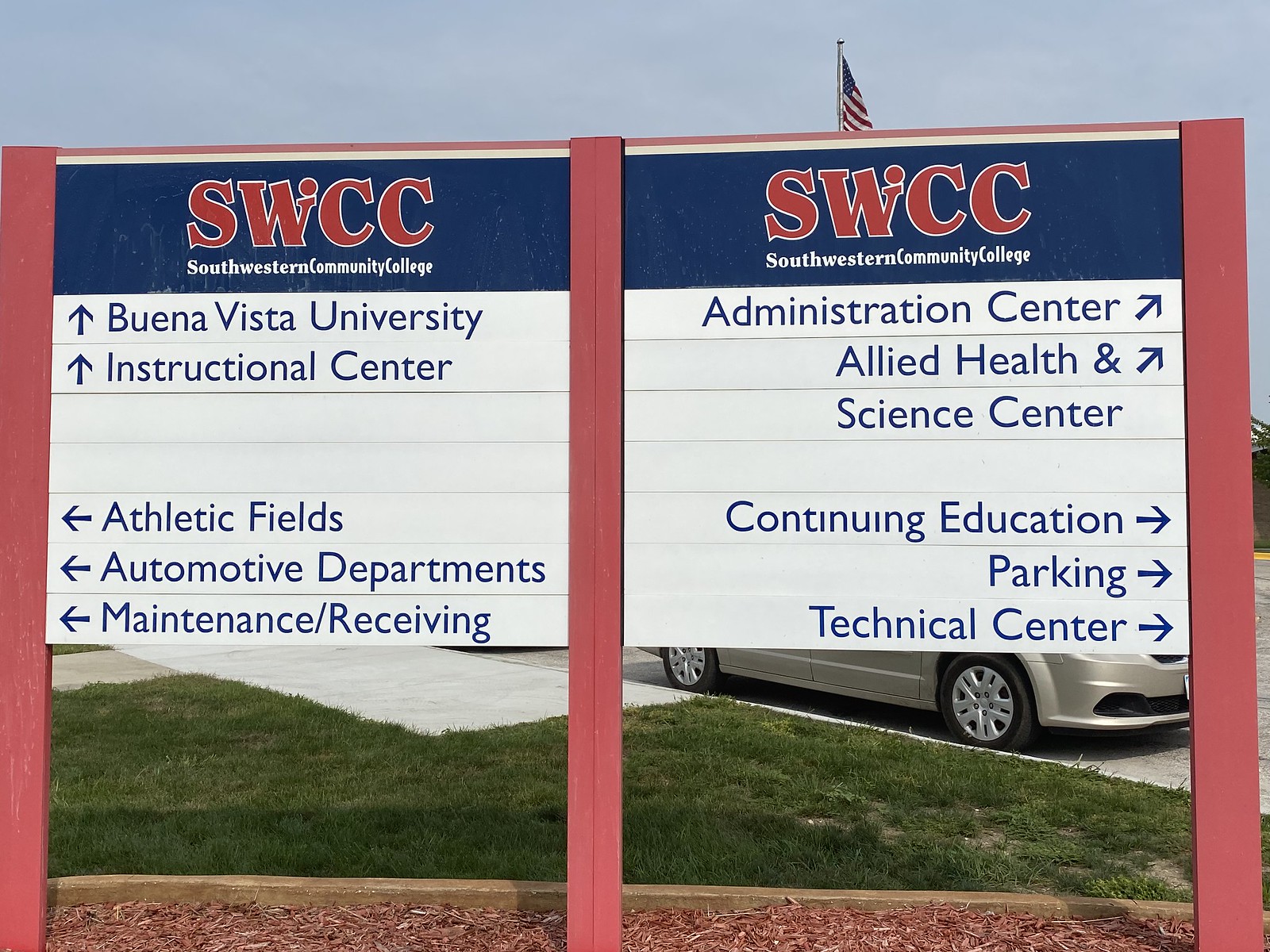This image features a detailed directional sign located at the center of a college campus setting, primarily dominated by Southwest Community College (SWCC) and its various facilities. The sign emerges from a mulch bed and contains blue and red markings directing to multiple destinations. At the top, “SWCC, Southwestern Community College” is prominently displayed, with subsequent directions: an arrow pointing straight to Buena Vista University and the Instructional Center. To the left, arrows indicate Athletic Fields, Automotive Departments, and Maintenance & Receiving. On the right side, arrows guide to the Administrative Center, Allied Health, Science Center, Continuing Education, Parking, and Technical Center. The background reveals a pastoral scene with a patch of green grass, a sidewalk, and a parking lot where a few vehicles, including what appears to be an older model car, are visible. Above, an American flag waves against the blue sky, adding to the serene midday atmosphere. The image vividly captures the organized layout typical of a well-maintained college campus.